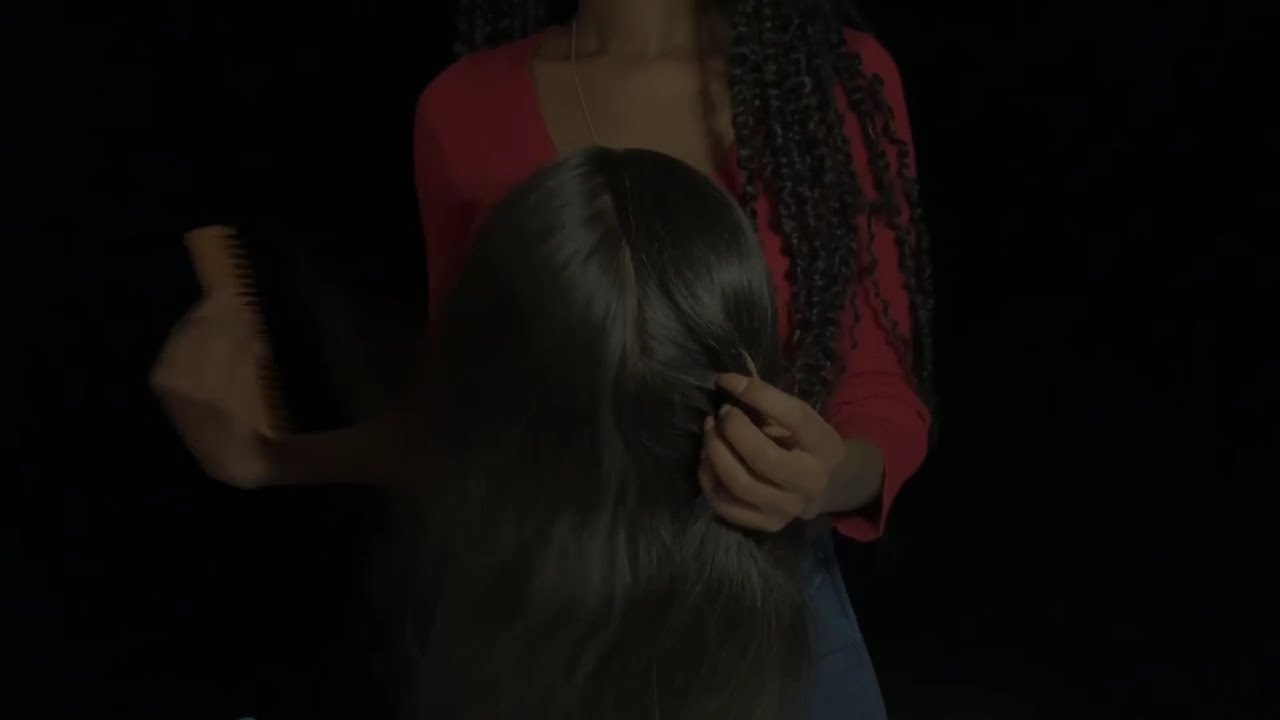In the center of a black background, a detailed photo captures a woman wearing a reddish-orange, long-sleeve sweater and blue Levi jeans, holding another figure close. The second figure, whose head is obscured as it faces the woman, appears to be a younger girl with long, smooth, dark hair. The woman’s hands, adorned with long nails, are gripping the girl's neck gently, suggesting a protective or affectionate embrace. The girl's hair looks freshly combed, as if just out of the shower, and she appears to have a navy-blue towel or sweater draped over her shoulders. The woman’s own hair includes a visible curly section coming down from her shoulder on the right, hinting at a ponytail or braid. The scene evokes a sense of intimacy against the stark contrast of the dark backdrop.